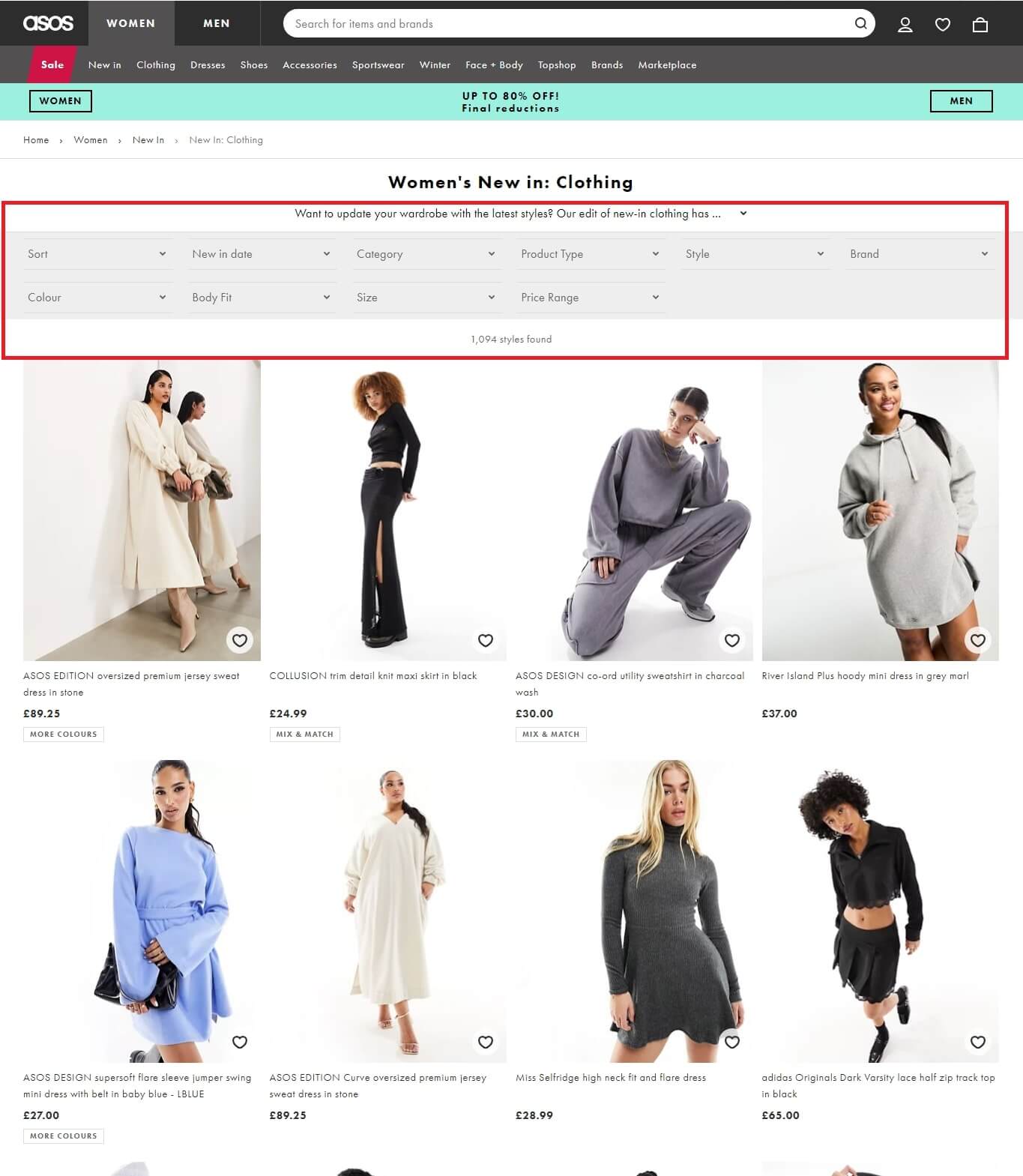**Detailed Caption:**

The image showcases a diverse selection of women's fashion available for purchase on ASOS, including new items and those on final reduction with discounts of up to 80%. The women depicted are modeling a variety of clothing options, illustrating the range of styles and categories offered. 

From left to right:
1. A woman gracefully poses in a long, elegant white gown.
2. Another woman showcases a sleek, all-black ensemble, pairing a stylish black shirt with a chic black dress.
3. A casual look is modeled by a woman in a cozy gray tracksuit.
4. Comfort and style merge as a woman sports a laid-back gray hoodie.
5. A woman in a vibrant blue short dress adds a pop of color to the lineup.
6. Dramatic and eye-catching, another model is pictured in a voluminous white dress.
7. A figure-hugging gray dress is perfectly displayed by a confident woman.
8. Lastly, a classic combination of a black shirt with a fashionable black skirt is worn by the final model.

The image captures the extensive variety of clothing ASOS offers, spanning from formal gowns to casual wear, all detailed with precision to emphasize fit, style, and versatility for the upcoming season.